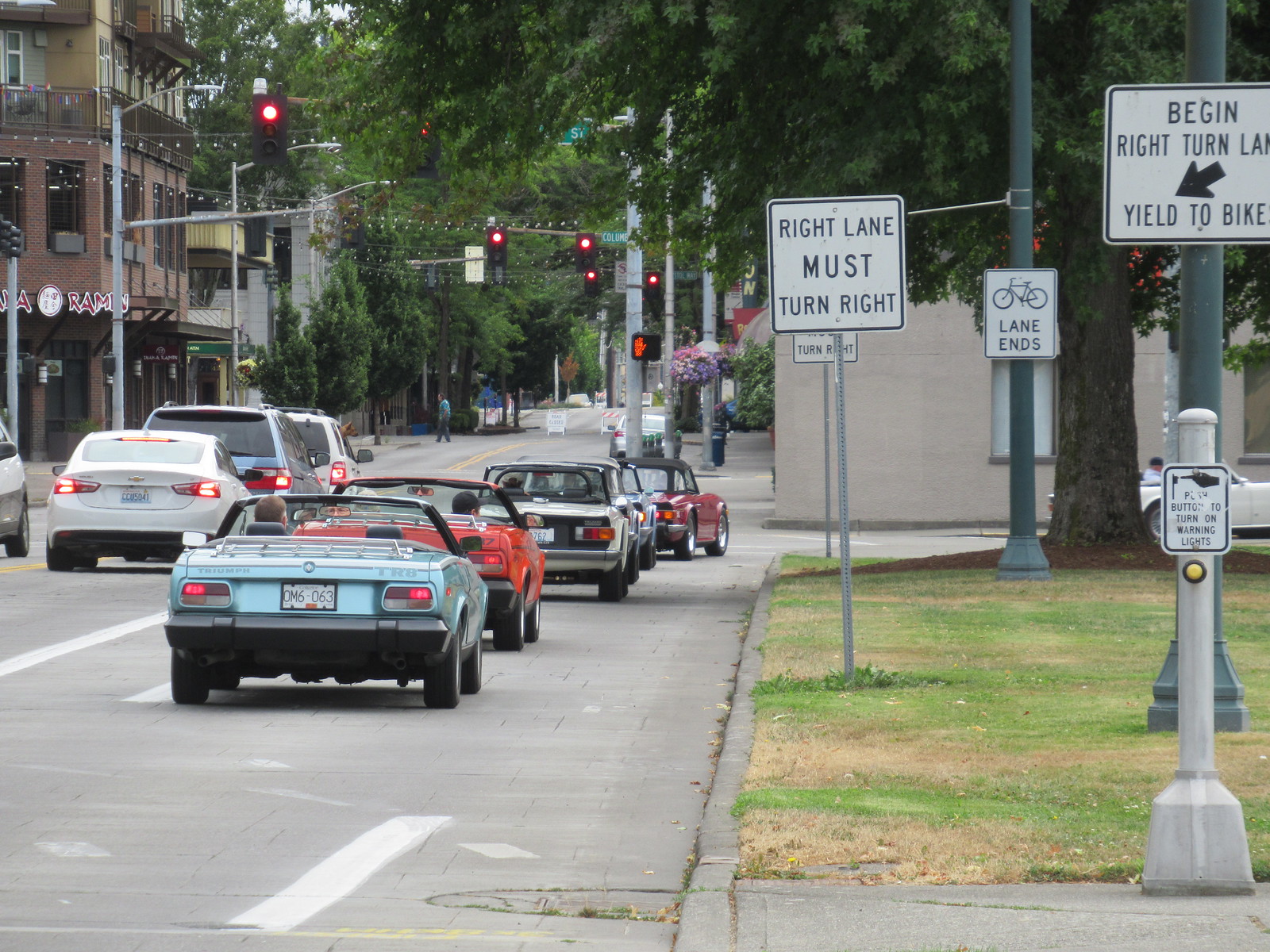The image depicts a bustling street in a metropolitan area. Buildings line both sides of the street, and a canopy of trees arches overhead, creating a tunnel effect. The street itself is marked by green pavement with white lane dividers. There are approximately seven to eight cars driving along, with the right lane exclusively occupied by convertibles in colors such as light blue, red, and white. Meanwhile, the left lane hosts a mix of many vans and a sedan in shades like maroon and gray. Red traffic lights hang over the street, halting all vehicles. 

On the right side, a grassy area borders the roadway, and several signs are visible, all affixed to green poles. One sign reads "Right Lane Must Turn Right," another indicates "Bike Lane Ends," and a third advises "Begin Right Turn Lane - Yield to Bikers." A fourth sign instructs pedestrians to "Push Button to Turn on Warning Lights." Notably, a large tree stands prominently on this side. On the left-hand side, there are additional buildings, including a ramen restaurant with a distinctive brick facade.